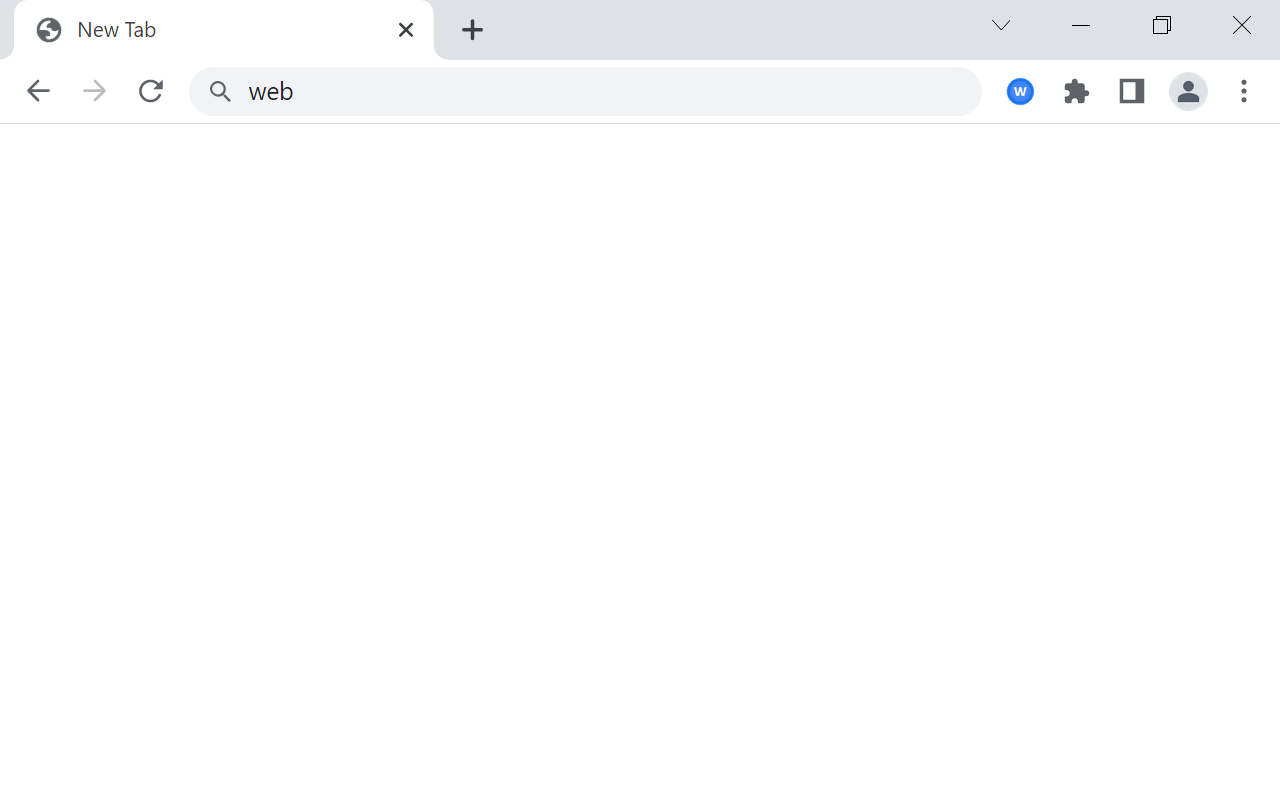The image is a screenshot of a blank browser tab on a Windows operating system. At the very top of the screenshot is the Windows bar, which is colored in light gray. On the left side of the tab bar, there is a tab labeled "New Tab" accompanied by a default globe icon. An "X" button is present to the right of this tab, which allows users to close it. Next to the tab, there is a plus (+) button for opening new tabs. Further to the right are icons for a drop-down menu, minimize, maximize, and close (X) functions.

Below the tab bar, there is the URL bar, which contains placeholder text that reads "web." On the far left side of the URL bar, there are navigation icons consisting of a back arrow, a forward arrow, and a refresh icon. On the right side of the URL bar, there is an icon of a "W" inside a blue circle, followed by an extensions icon represented by a puzzle piece, a square icon likely representing an app or additional feature, a profile icon set to a default avatar, and a three vertical dots icon for additional browser options.

The main area of the browser window displays a completely blank page with a white background.